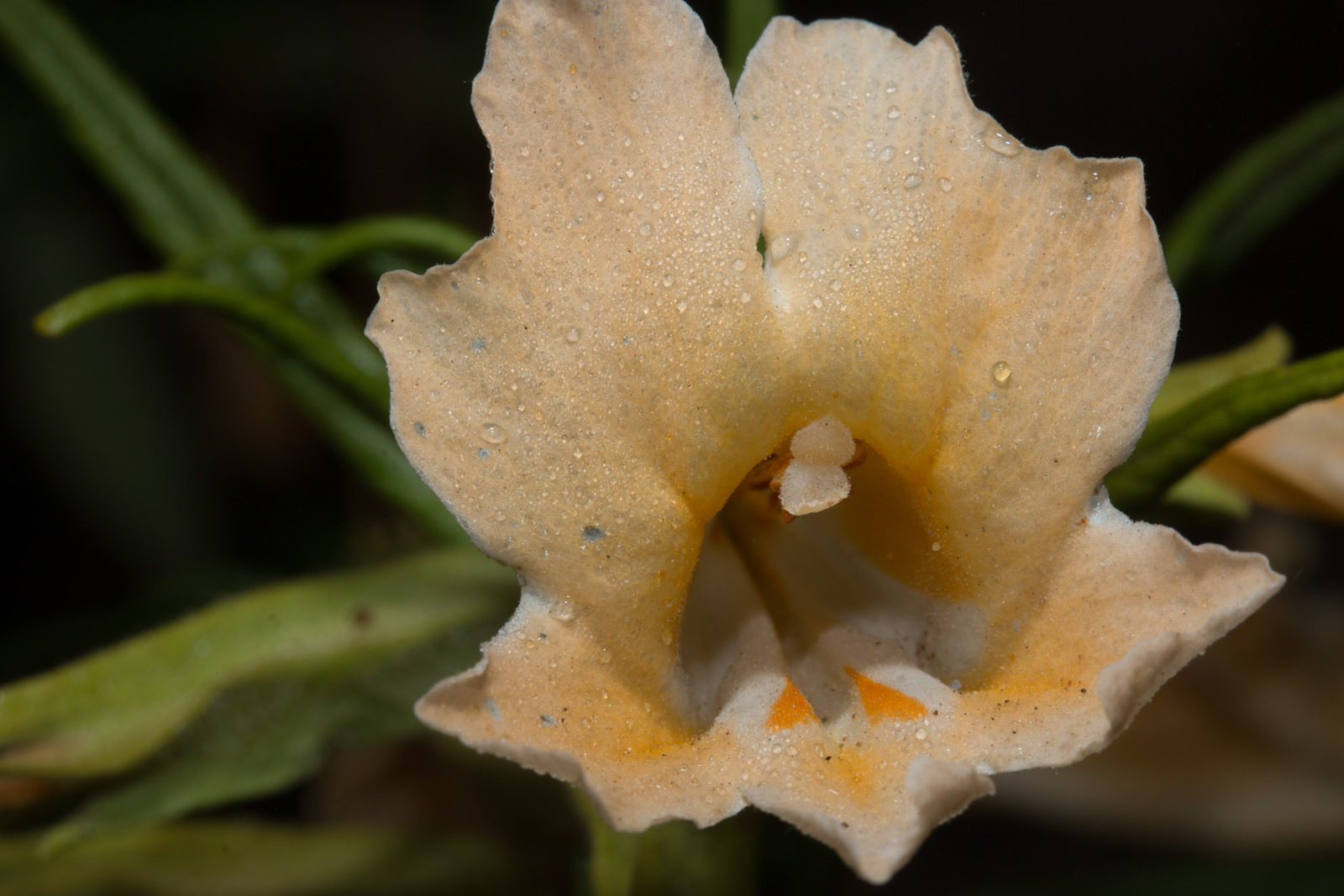This is an incredibly detailed macro photograph of a flower, possibly a type of lily, capturing its intricate beauty in a portrait view. The flower dominates the center from top to bottom, displaying its open petals in a blend of light orange, peach, and dark white hues. Delicate water droplets are scattered across its surface, glistening in the light. The interior of the flower is strikingly white, with vibrant orange triangular sections adding contrast. The very center contains two white stamens, poised to hold pollen.

The background is a deep, almost black darkness, suggesting this photo may have been taken at night or with significant shadowing. Various green leaves frame the flower from different corners – the top left corner features a distinct green leaf, the top right has a touch of green against the black, the bottom left corner has bright to dark green leaves slightly faded, and the bottom right has darker shades, possibly purples and grays. The lush greenery surrounds the flower, enhancing its vibrant colors and the immaculate details of this close-up shot.